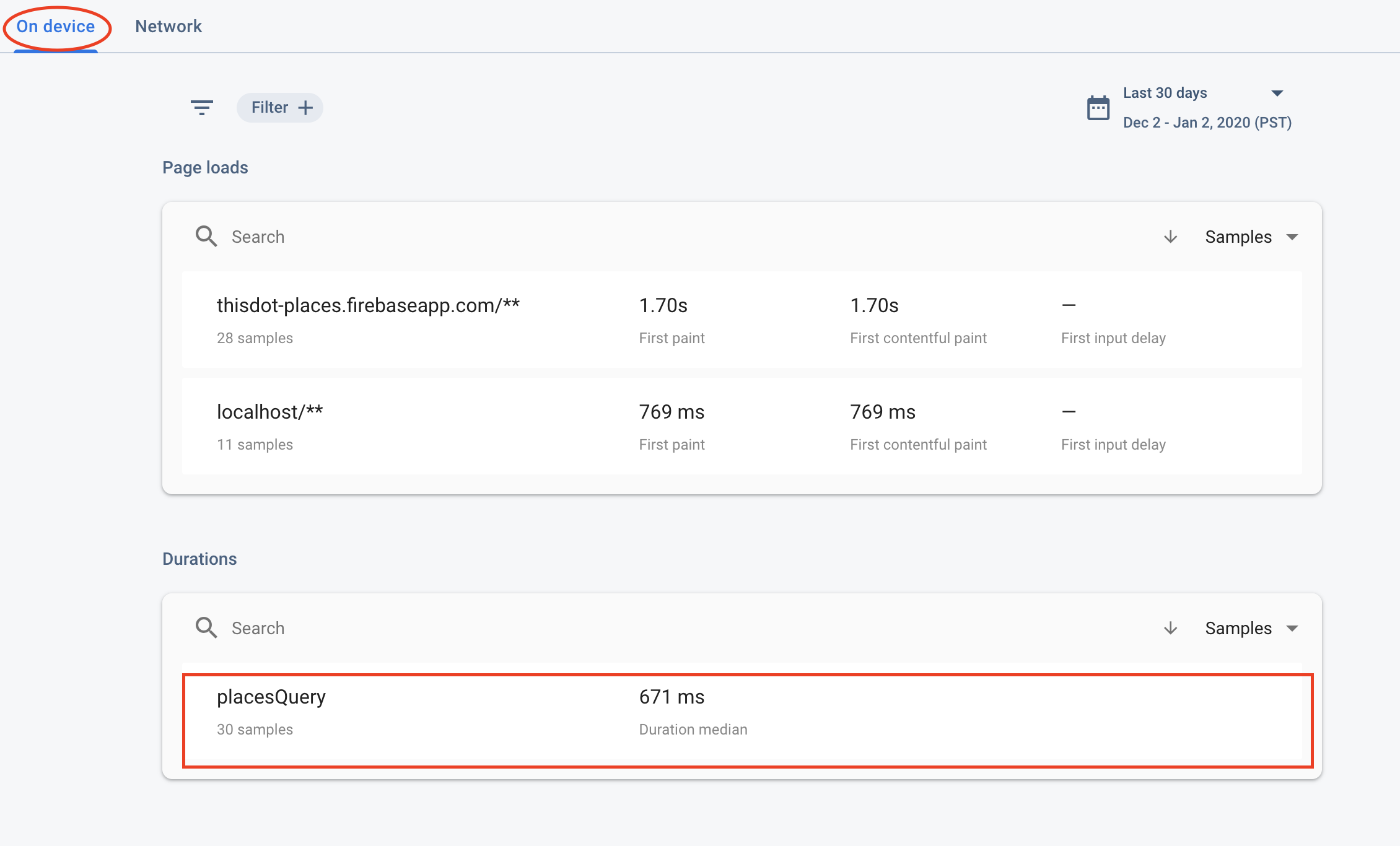Here's a comprehensive and cleaned-up caption for the image:

---

This edited screenshot provides a detailed view of a tutorial interface focused on performance metrics. At the very top of the image, two options are available: "On Device" and "Network". The "On Device" option is currently selected, as indicated by the red oval line encircling it. 

Directly below these options, the interface is divided into two main sections: "Page Loads" and "Durations". In the "Durations" section, there is an entry labeled "Query Results", with "30 samples" noted beneath it. To the right, the metric "671 ms" (milliseconds) is displayed, with a label "Duration Median". This entire row is highlighted with a red box. 

Additionally, there is a sorting option to the right, labeled "Samples Sorting", suggesting that users can organize the data based on different criteria by selecting this option. Both the "Page Loads" and "Durations" sections come with a search functionality, giving users the ability to filter results.

In the "Page Loads" section, two URLs are presented: "dot-dash.places.firebaseapp.com/**" and "localhost/**", indicating specific pages or endpoints being analyzed.

---

This caption is detailed, providing clarity on what each part of the screenshot represents and the significance of the highlighted features.